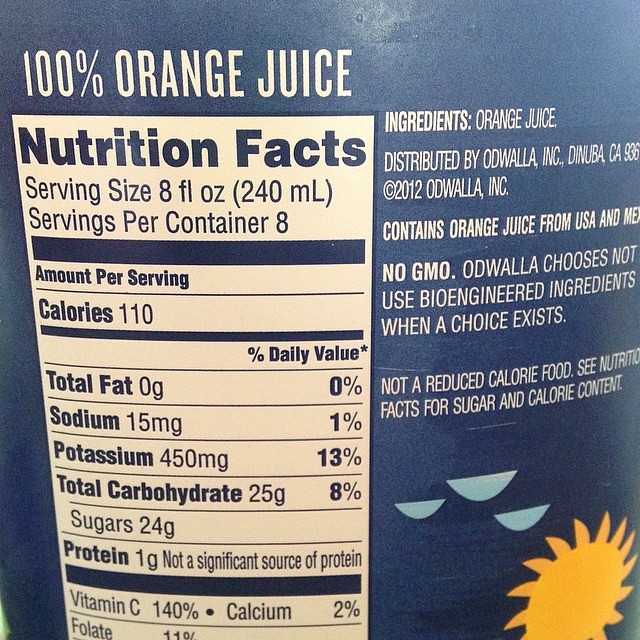This image features a blue container of orange juice prominently displaying its nutritional facts and ingredients. The container showcases a vibrant blue background with white lettering. The nutrition label provides key information as follows: 

- Serving size: 8 fluid ounces
- Calories per serving: 110
- Total fat: 0 grams
- Sodium: 15 milligrams
- Potassium: 450 milligrams
- Total sugars: 25 grams
- Protein: 1 gram

Notably, the juice is not a significant source of protein and is labeled as non-GMO and not a reduced-calorie food. The juice contains 140% of the daily recommended value of Vitamin C, 2% of calcium, and 11% of folate per serving.

The ingredients list, positioned next to the nutrition facts, confirms that the product contains 100% orange juice. The container also features a sun design and water droplets, enhancing its fresh and natural appeal. The combination of bright blue and white ensures the information is easily readable against the backdrop.